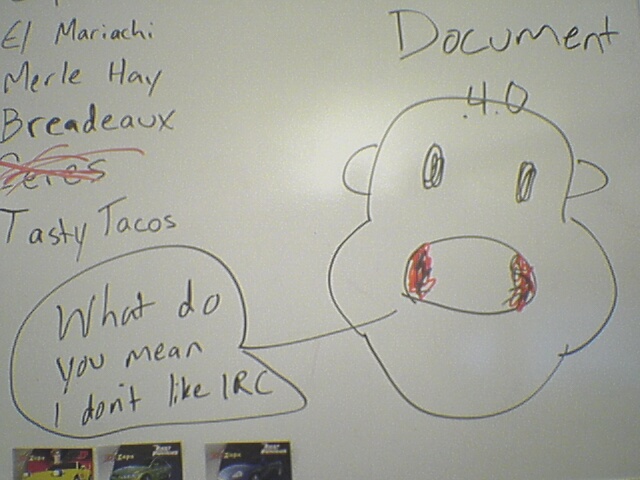The image is a detailed and somewhat chaotic drawing on a white piece of paper, resembling a child's doodle or scribbles. The top right corner prominently features the handwritten text: "Document 40." Below this, there's a drawing of a head, more sophisticated than a simple smiley but not highly realistic, with an open mouth speaking. A speech bubble to the left of the head contains the text: "What do you mean I don't like IRC?" Scattered around the top left corner are the words "El Mariachi," "Merle Hay," "Bredo," and "Tasty Tacos." Additionally, there's a crossed-out phrase, possibly "series" or "zeros," marked in red. On the drawing, three fuzzy, indistinct rectangles positioned somewhere suggest images of cars in yellow, green, and blue colors, but details on these are unclear. The overall appearance is as if it's been done on a dry-erase board, though it's on a piece of paper.